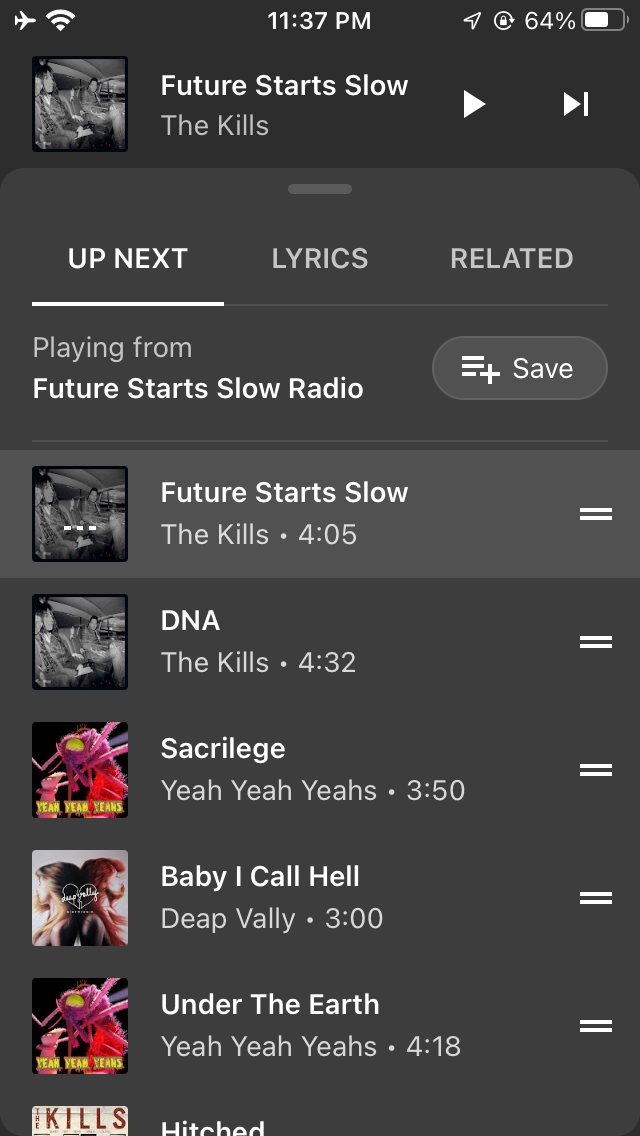This image appears to be a screenshot taken from an iPhone at 11:37 PM with the battery level at 64% and the device in airplane mode, yet still showing a strong connection. The top black bar reads "Future Starts Slow," a song by The Kills, with a white arrow pointing to the right. Adjacent to the arrow is a white box with another white arrow. Below this bar, a black and white album cover can be seen next to the text "Up Next," "Lyrics," and "Related," with "Up Next" highlighted by a white underline. The section states that the song is playing from "Future Starts Slow Radio" and includes a gray "Save" button. Listed below are several song titles and artists including:

1. "The Future Starts Slow" - The Kills
2. "DNA" - The Kills
3. "Sacrilege" - Yeah Yeah Yeahs
4. "Baby I Call Hell" - Deap Vally
5. "Under the Earth" - Yeah Yeah Yeahs
6. "Hitched" (partial details cut off)

The image cuts off further details beyond this list.